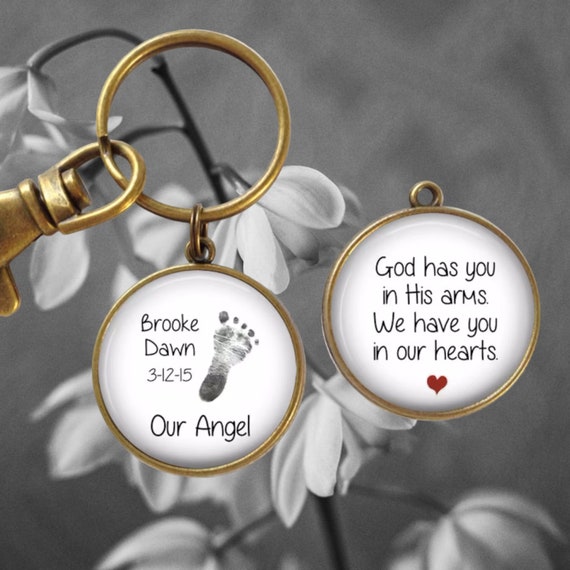The image shows a delicate locket-style necklace design with two pendants set against a black-and-white backdrop of drooping flowers. A golden carabiner, coming from the left-hand side, secures a circular gold ring attaching the left pendant. This pendant displays the words "Brooke Dawn 3-12-15 Our Angel" alongside a tiny footprint. The second pendant, positioned to the right on a white background, features a red heart at the bottom and the black-printed message "God has you in his arms, we have you in our hearts." The combination of the detailed gold pendants and the monochromatic floral background gives the image a poignant and heartfelt appearance.